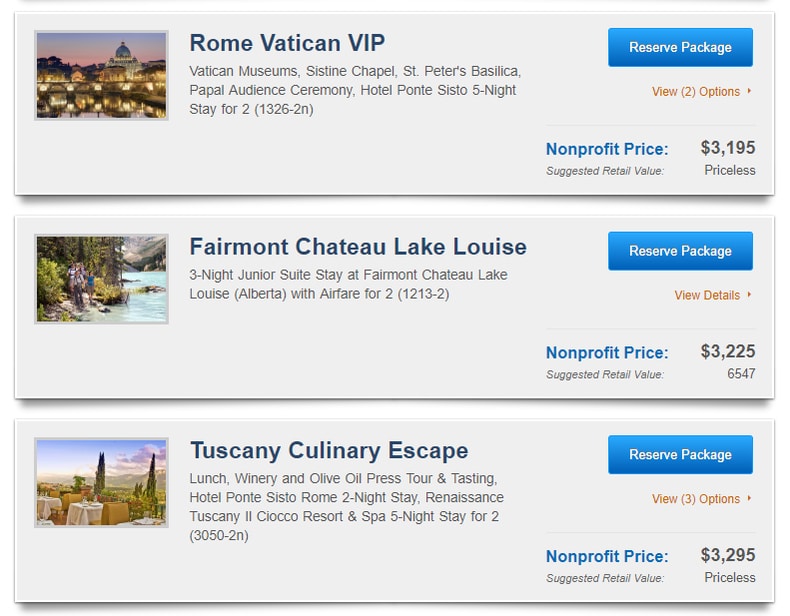This image showcases three distinct tourist attraction packages available for reservation. At the top, the "Rome, Vatican VIP" package includes visits to the Vatican Museum, Sistine Chapel, St. Peter's Basilica, and a Papal Audience Ceremony. It also offers a five-night stay for two at the Hotel Ponte Sisto. This package is priced at a non-profit price of $3,195, though its suggested retail value is deemed priceless. A gold-lit distant building contrasts beautifully with a pink and purple sky, enhancing the top-left corner of the image. The call-to-action "Reserve Package" is prominently displayed in blue, with options to view details and the non-profit price starting at $3,195.

The second package, "Fairmont Chateau Lake Louise," features an image of a serene lake surrounded by lush trees. This package offers a three-night junior suite stay at Fairmont Chateau Lake Louise in Alberta, paired with airfare for two. The reserve package price is set at $3,225, while its suggested retail value is $6,547.

The third offering, titled "Tuscany Culinary Escape," is represented by an image of picturesque natural scenery. To the right, the details mention a reserve package with a non-profit price of $3,295.

Each of these exclusive packages presents unique travel experiences, highlighting cultural landmarks, luxurious accommodations, and natural wonders.